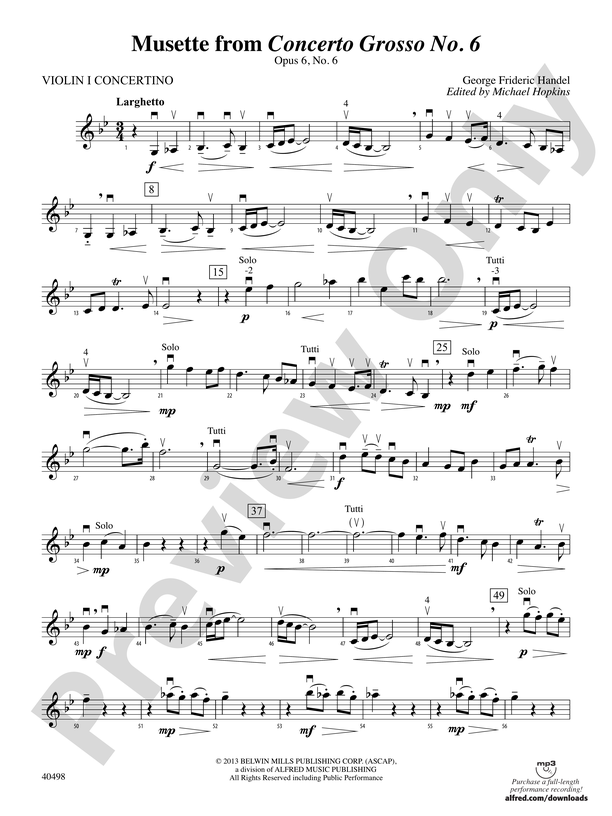The black and white image features a piece of sheet music in portrait orientation with the title "Musette from Concerto Grosso No. 6" prominently displayed at the top. Underneath the title, in smaller text, is "Op. 6 No. 6." It is designated for "Violin I, Concertino" on the top left-hand corner, indicating the instrument part. On the top right-hand side, the composer is identified as "George Friedrich Handel," with editing credits to "Michael Hopkins" in italicized text. The sheet showcases about ten lines of music, all in the treble clef, with notes, rests, and key changes meticulously notated. Towards the bottom center, the copyright information reads "2013 Bellwin Mills Publishing Corp., Forensics ASCAP," accompanied by an illegible logo on the bottom right. A unique identifier, "40498," is noted at the bottom left. A diagonal watermark stating "Preview Only" spans across the music from the bottom left to the upper right corner.